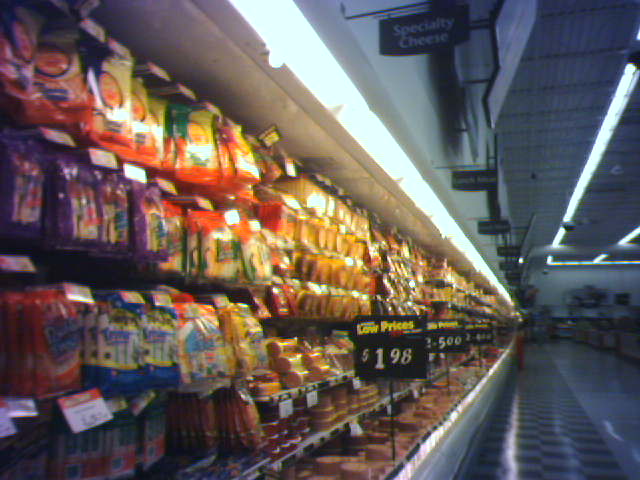This photograph captures the cheese and deli section of a grocery store, showcasing a long refrigerated cooler that spans nearly three-quarters of the aisle length, filled with various packaged cheeses and lunch meats. The cooler is illuminated by fluorescent lights, which highlight an assortment of colorful packaging in yellow, green, purple, and blue. In the midsection of the cooler, numerous black signs on sticks display price tags and sales information, such as signs indicating "Low Prices" with a visible price of "$1.98."

The ceiling above features exposed rafters and long fluorescent lights, typical of a warehouse-style setup, giving the impression of an open, industrial feel. The backdrop includes a white wall adorned with a black sign reading "Specialty Cheese." The floor at the bottom right of the image is a mix of solid gray and a checkered pattern, slightly out of focus. The overall ambiance suggests a mom-and-pop grocery store rather than a large chain, emphasizing a more personal shopping experience in a specialized cheese and deli section.